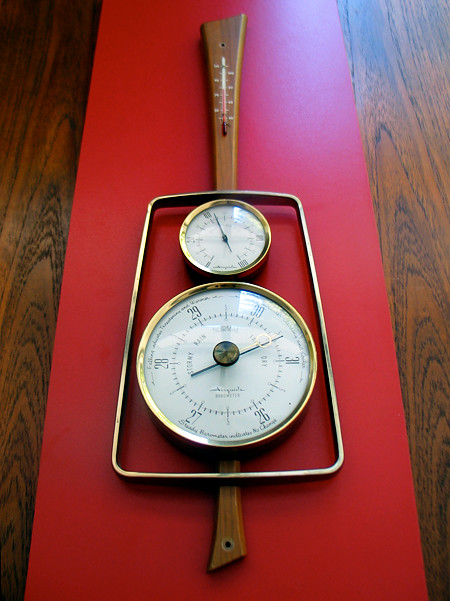This vertically oriented photograph captures a scene set on a dark reddish-brown wooden table. Dominating the background is the table's rich texture. Running down the center of the image is a red strip, which appears to be part of a box or platform of some kind. Resting on this red strip is a striking, ornate tool. The tool features a long, slender wooden neck, and at its top is a built-in thermometer. Midway down the tool, there is a metal frame with a hollow center that houses two round dials. These dials, akin to clock faces, have white interiors marked with black numerals and dials, suggesting they measure air pressure or temperature. The detailed craftsmanship of the instrument and the intricate dials lend the photograph a sense of curiosity and precision.